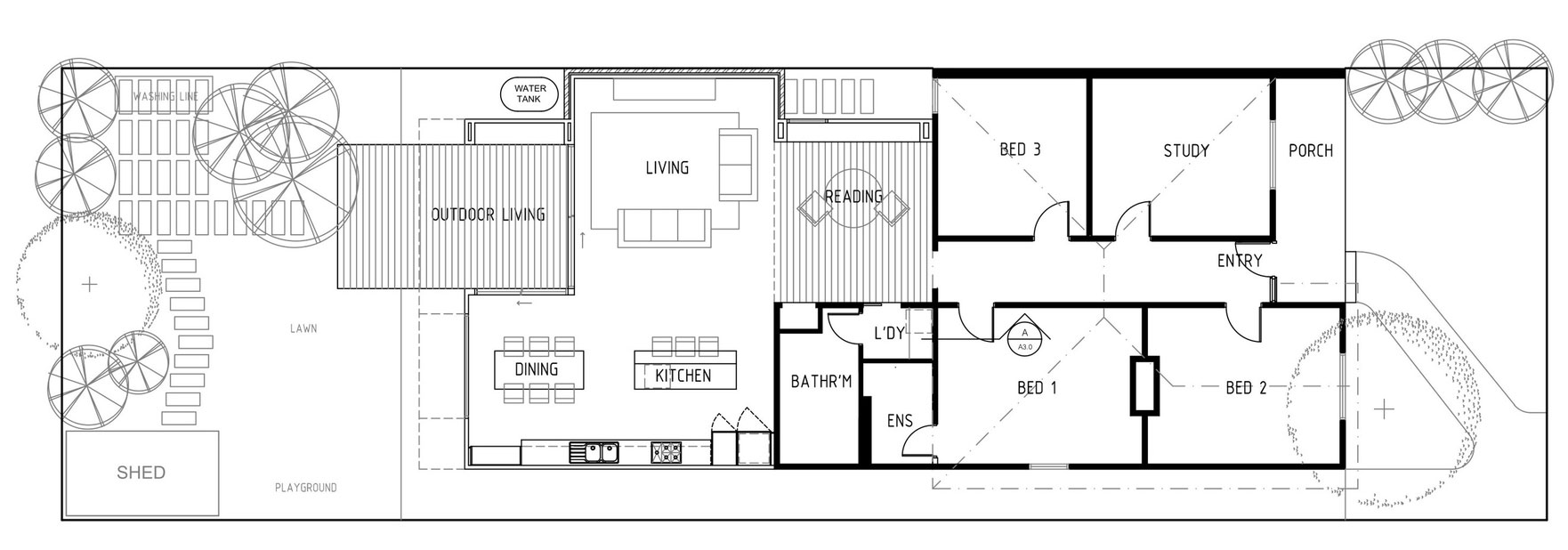This image is a detailed floor plan of a house, depicted with a distinct black outline. Starting from the top right, there are two drawn circles. The layout begins with a porch at the entrance. Adjacent to the porch is a square room designated as a study. Next to the study is another square room labeled "Bed 3." Moving through a hallway that stretches from the bottom to the right, the bottom-right square room is labeled "Bed 2." Beside that is "Bed 1," also a square room.

Following the bedrooms, there is a smaller room marked "Ens" (en suite bathroom) and another small room labeled "Ldy" (laundry). The next room is the bathroom. Above these rooms is an additional space characterized by lines and labeled "Reading."

To the left of the "Reading" area is a larger room labeled "Living," and below that, a space designated as the "Kitchen." To the left of the kitchen is the "Dining" room. Above the dining room, there's a large square area with lines through it, labeled "Outdoor Living," which leads to the backyard area.

The backyard itself features numerous drawn circles, possibly indicating landscaping elements, and includes a square labeled "Shed."